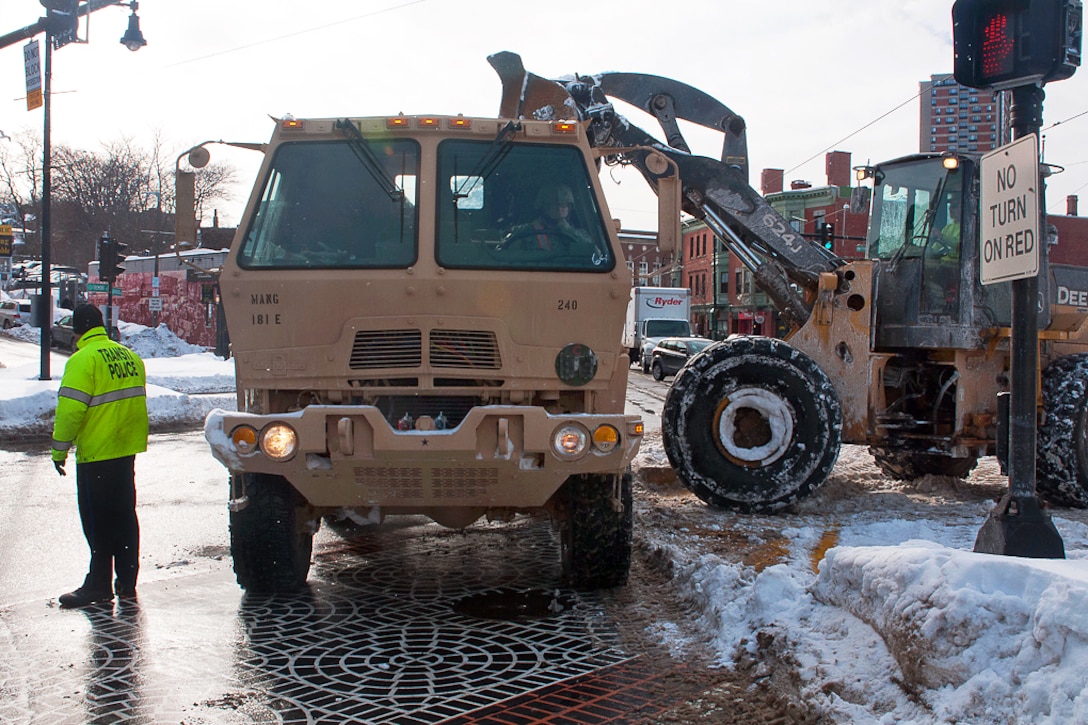This image depicts a bustling scene in a small town square on a snowy winter morning. Central to the photo is a yellow dump truck facing the camera, with its driver visible in the cockpit. A backhoe is actively loading material into the truck's bed, though the exact contents remain obscured by the cab of the dump truck. To the left of the image, a transit police officer wearing a fluorescent jacket and black pants is seen directing traffic. His jacket clearly reads "Transit Police" in black lettering. Adjacent to him is a streetlight with a "No Turn on Red" sign and a pedestrian signal indicating 'don't walk'. The environment is characterized by a significant amount of slushy, muddy snow on the ground, hinting at recent clearing efforts. In the background, the town's charm is accentuated by red brick buildings and a parked Ryder rental truck. Overall, the image captures a moment of coordinated activity amidst the wintery setting, with the transit police ensuring safety and smooth operation as the backhoe and dump truck carry out their tasks.